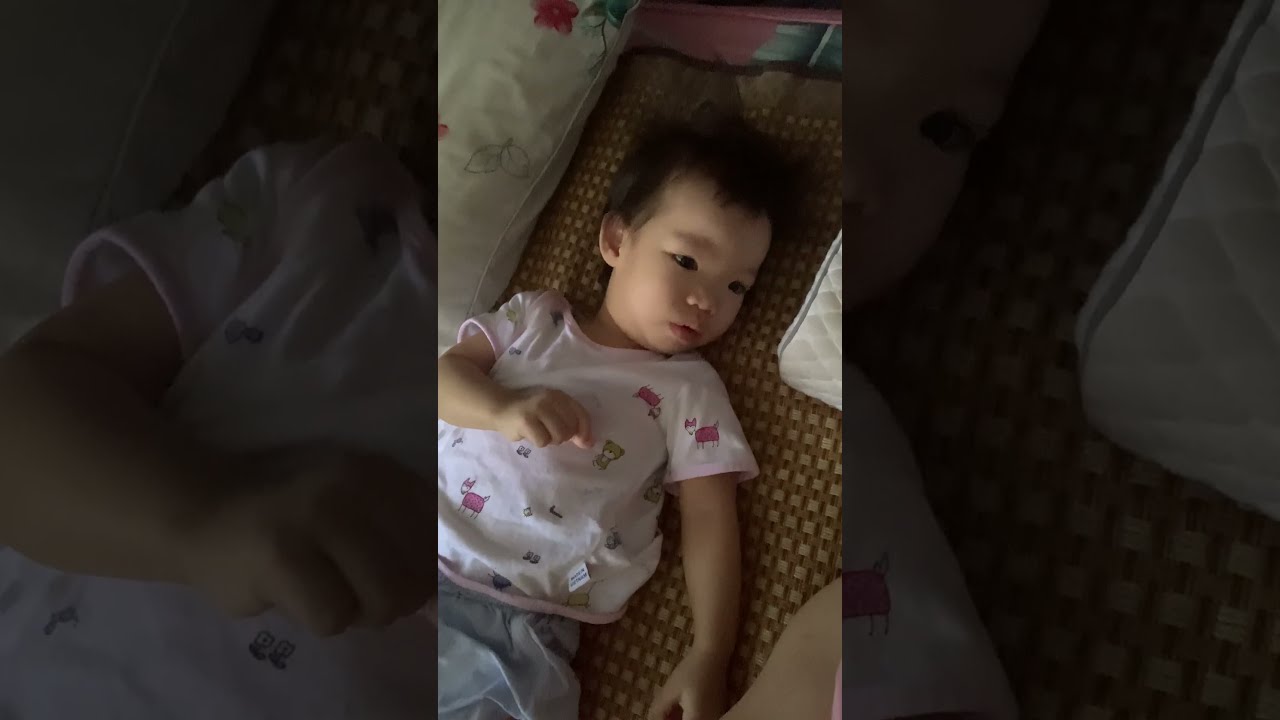In a cozy bedroom or living room setting, a photographic image captures an Asian toddler girl lying on her back on a brown and tan interwoven checkerboard-patterned rug. She wears a pink shirt adorned with various little cartoon animals, including cats and teddy bears. The child has dark hair and dark eyes, and her facial expression is engaged, as she gazes off to the right. One of her arms rests on her chest, while the other lies on the floor beside her. The background features a wall with a green-gray plant and a red flower. The photo emphasizes the central panel, with the left and right panels blurred out, bringing the girl into sharp focus. A floral pillow and a folded quilt are also seen near her, adding to the cozy atmosphere.